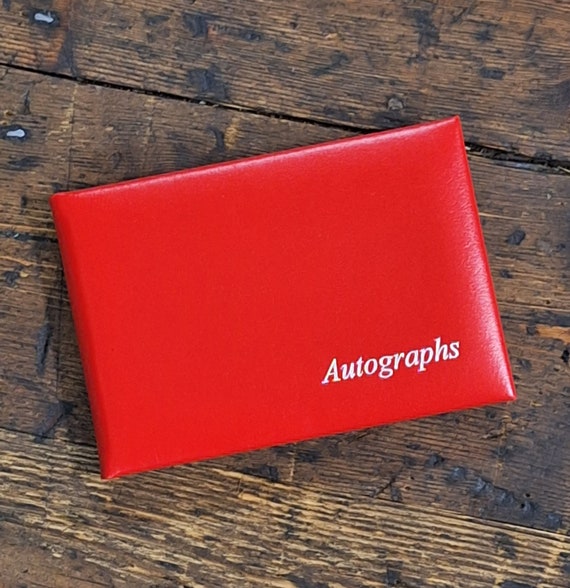This photograph showcases a vibrant red, patent leather autograph book, adorned with the word "autographs" emblazoned in white lettering on the bottom right-hand corner. The book, in pristine condition, catches the light, highlighting its glossy finish. It rests against a rustic, homemade wooden table, notable for its dark brown hue, burn marks, and a few lighter scrape marks, adding a nostalgic touch to the setting. The table's aged appearance contrasts sharply with the book's vibrant red, making it stand out. Positioned slightly askew, the book tilts downward on the left and upward on the right, suggesting a casual yet deliberate placement. The overall composition and sharp details of the image aptly capture the essence and condition of the autograph book, making it an excellent representation of this historical keepsake.